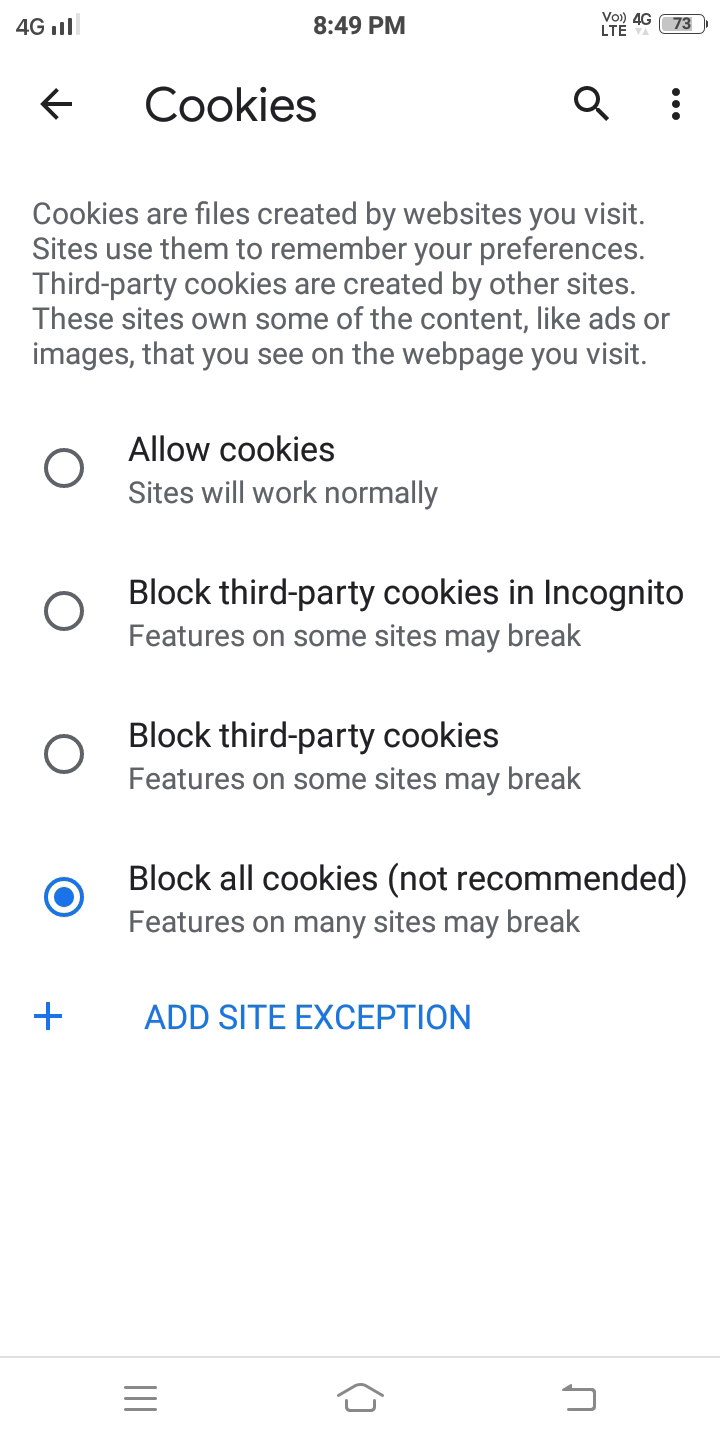The screenshot shows a device interface set against a solid white background. 

In the upper left corner, the status indicators are displayed, showing "4G" and signal strength with 3 out of 4 bars in black text. The current time, "8:49 PM," is centered at the top, and a battery icon with "73%" is visible in the upper right corner.

Below the status bar, the word "Cookies" is displayed prominently in large black text. To the left of "Cookies," there is a left-pointing arrow icon, and to the right, there is a magnifying glass icon, indicating search functionality.

Underneath, in gray text, it describes:
"Cookies are files created by websites you visit. Websites use them to remember your preferences. Third-party cookies are created by other sites. These sites own some of the content, like ads or images, that you see on the web page you visit."

Following this informational text, bold text reads:
"Allow cookies."

An explanatory note below states:
"Sites will work normally."

Further down, another option in bold text reads:
"Block third-party cookies in incognito."

Underneath that, there is a warning:
"Features on some sites may break."

Finally, another bold black text option:
"Block third-party cookies."